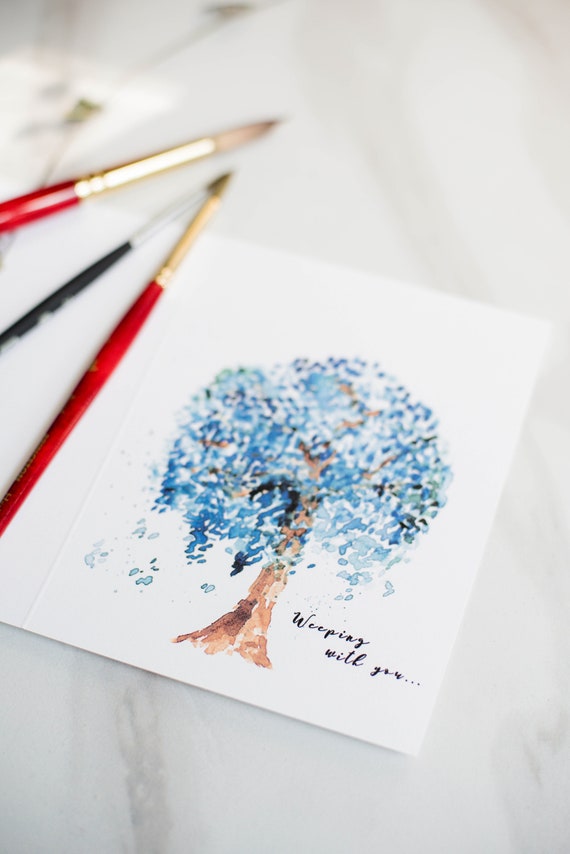This photograph captures a top-down view of a delicate watercolor painting on a card, positioned on a white marble tabletop. Central to the image is a stylized tree with a bright brown, solid trunk and a voluminous canopy of blue and dark blue leaves, suggesting the likeness of a weeping willow. Beneath the tree, some leaves are illustrated falling, adding to its expressive nature. In the bottom-right corner of the card, there's black text reading, "weeping will you..." hinting both at the tree's type and perhaps a deeper message. To the top left of the card, three fine-tipped watercolor brushes are arranged in a triangle, their handles painted in distinct colors—red, black, and dark red. This scene is richly colored, featuring predominantly white, gray, blue, brown, and red hues.